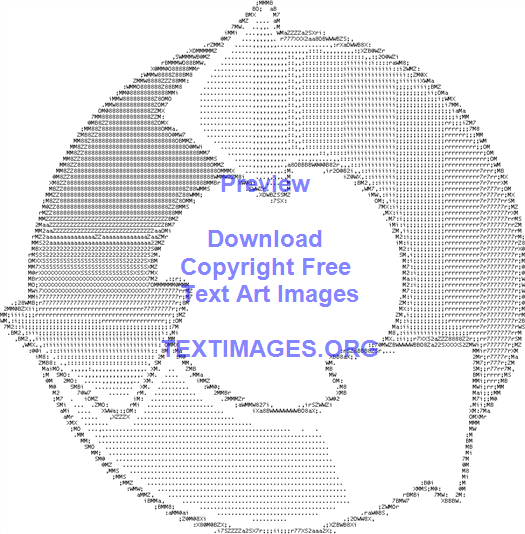The image is a grayscale graphic featuring three overlapping circular arrows forming a loop, arranged to create a cohesive circle. The arrows point counterclockwise: the first arrow starts at the bottom right with a pale shade, progressively darkening as it curves to the left and upwards; the second arrow, positioned at the top, has about three-quarters of its point dotted with letters and numbers, reminiscent of old dot matrix printer text; and the third arrow, curving back downward, is fully detailed with similar dot matrix-style elements. In the center of this circular design, printed in light purple text, are the words "Preview," followed by "Download," "Copyright-Free," "Text Art Images," and at the bottom, in all caps, "textimages.org." The entire graphic is set against a plain white background, with no additional images or text present, emphasizing the intricate design and textual details within the arrows.